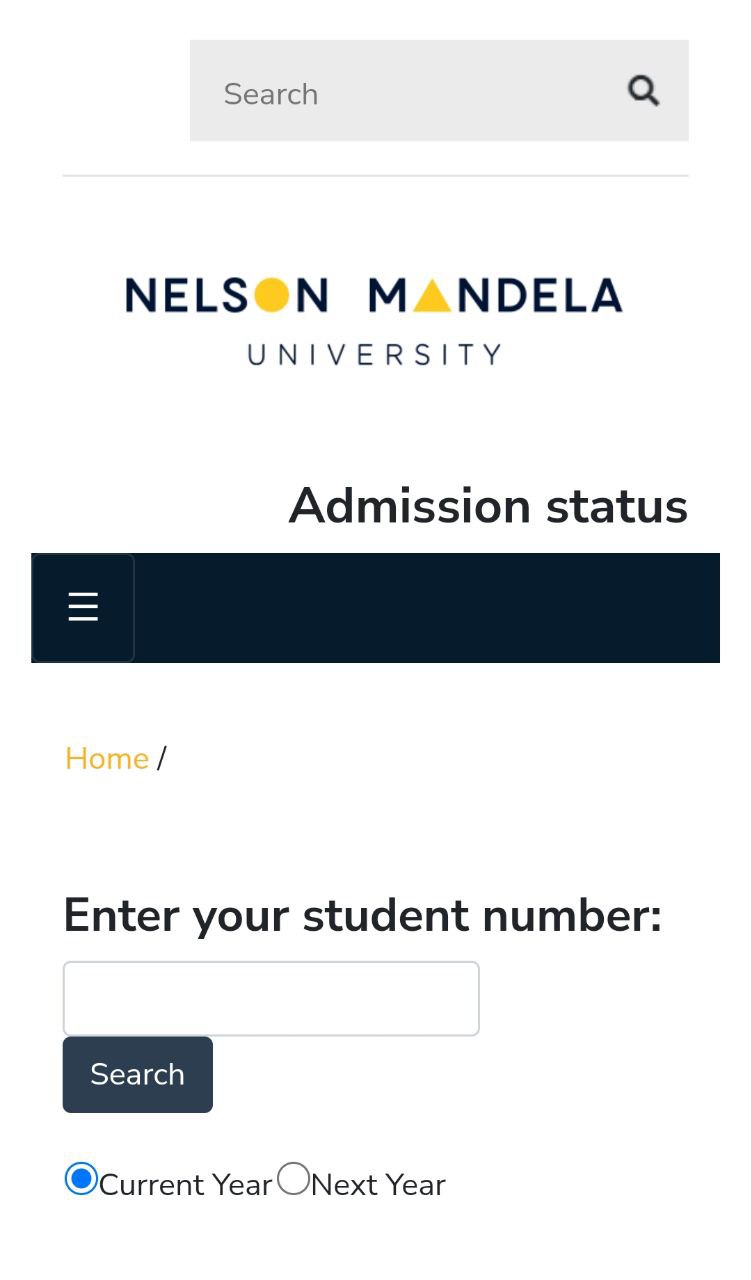The image depicts a search page for Nelson Mandela University. At the top of the page, a gray search bar is prominently displayed. Directly beneath this bar, the page header shows the text "Nelson Mandela University," where the letter 'O' in "Nelson" is creatively replaced with a yellow circle, and the first 'A' in "Mandela" is substituted with a yellow triangle.

Below the university name, the text "admission status" is clearly visible. This is followed by a black navigation bar featuring three horizontal lines on the left, indicating a menu. Directly beneath this bar, the word "Home" appears in yellow, accompanied by a forward slash.

Further down the page, instructions prompt users to "enter your student number," followed by an input box for the student number entry. Below this input box is a "Search" button. Additionally, there is an option to select the admission status for either the current year or the next year, with the current year option highlighted.